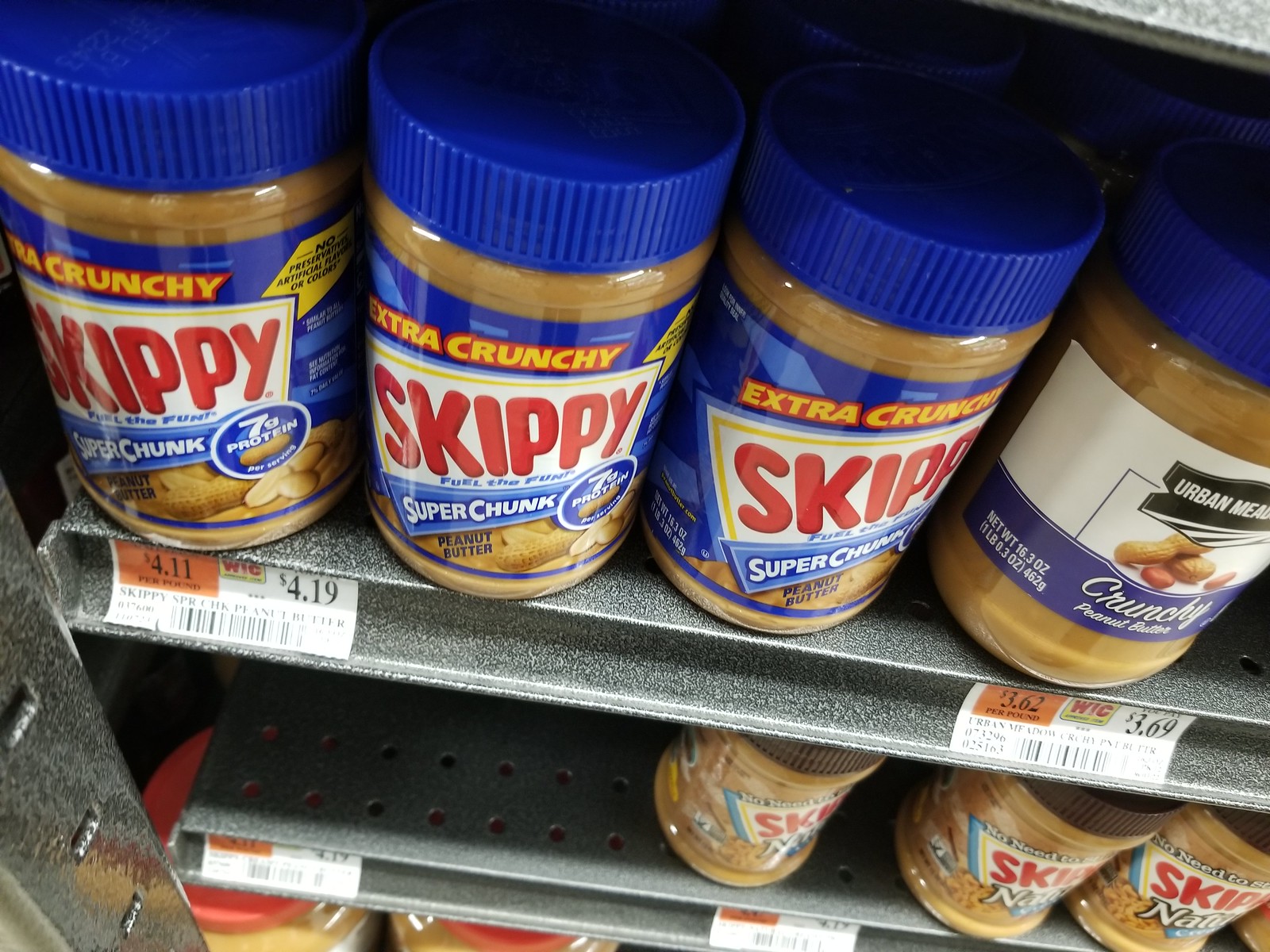The image depicts a zoomed-in view of a grocery store shelf dedicated to peanut butter jars, showcasing multiple rows and brands. The top shelf prominently features four jars, the first three being Skippy Super Chunk with extra crunchy peanut butter, identified by their blue lids and distinctive blue labels with "Skippy" printed in red on a white background. Next to these is an Urban Menu crunchy peanut butter jar, characterized by its more generic look with a white label and blue lid. The pricing tags below these jars indicate $4.19 for the Skippy jars and $3.69 for the Urban Menu jar.

Beneath the top shelf, another row of peanut butter jars is visible, including Skippy Natural, suggested by their brown lids and partially obscured labels with the letters "NAT" in white and a similar red "Skippy" logo. The price tag for this variety indicates $4.17. On the bottom shelf, there are larger jars of peanut butter with red lids, though the brand and specific type are not discernible due to the limited view.

The entire assembly is supported by steel shelving units, with square metal pipes and perforated sides for attaching the shelves. The white pricing tags prominently feature boxes in orange, marking different prices as $4.11, $4.19, $3.62, and $3.69. The overall setup is indicative of a well-organized store display, focused on providing clear visibility and pricing for the various peanut butter products.